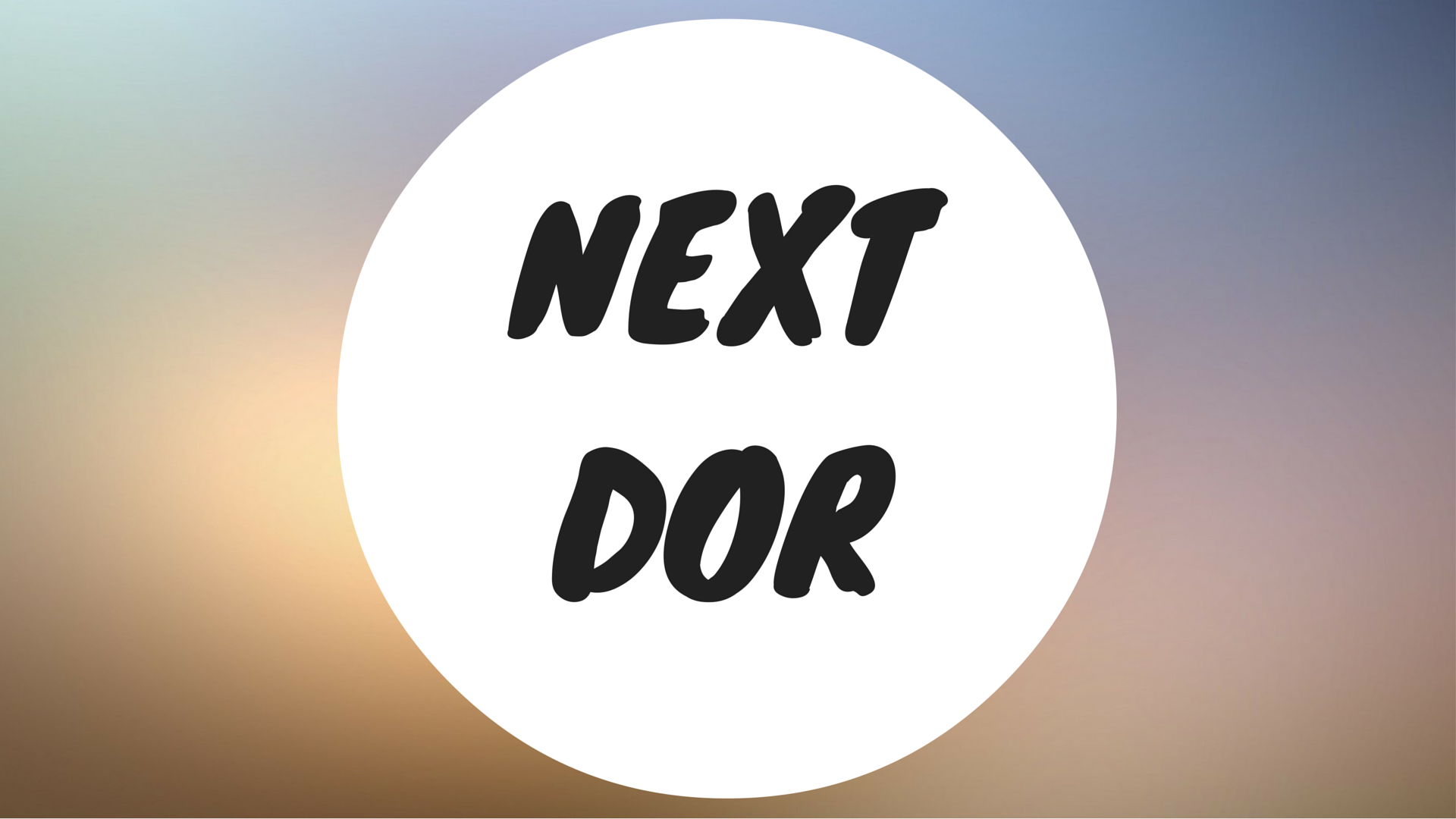The image presents a surreal, digitally edited scene dominated by a blurred and colorful background, featuring a gradient mix of navy blue, brown, green, pink, yellow, beige, and black. In the dead center of the image, a large, solid white circle holds the focal point. Inside this circle, bold, black text in a brushstroke style reads "Next" above "DOR" (not the conventional "DOOR"), with "Next" on top and "DOR" directly beneath it. The background outside the circle remains intentionally out-of-focus, drawing the eye directly to the central text within the crisp, white circle.